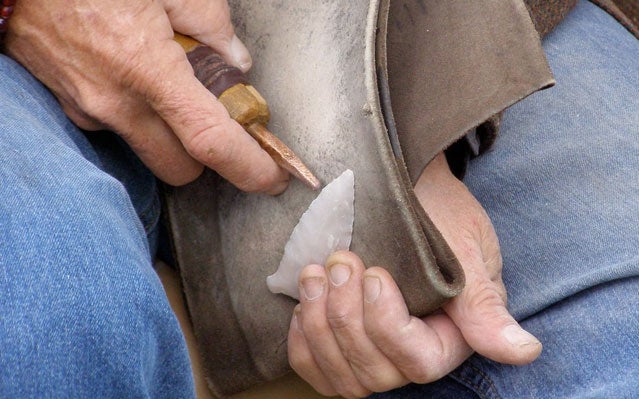The image features an older man with weathered, slightly wrinkled hands and short fingernails, intensely focused on working with a tool on a piece of leather. His blue jeans are visible on either side of the image, framing his lap where the action is centered. He holds a brown, folded piece of worn leather in his left hand, while his right hand grips a tool with a brown leather-wrapped handle and a metal tip that comes to a slanted, dull point. The tool resembles a screwdriver and appears to be pressing into the leather. At the tips of his right fingers is a peculiar grayish-white object that looks like an arrowhead, placed strategically against the leather. The entire scene reflects a close-up view, showcasing not just the tools and materials but also the careworn details of the man’s hands and attire, suggesting a deep involvement in a meticulous leatherworking task.